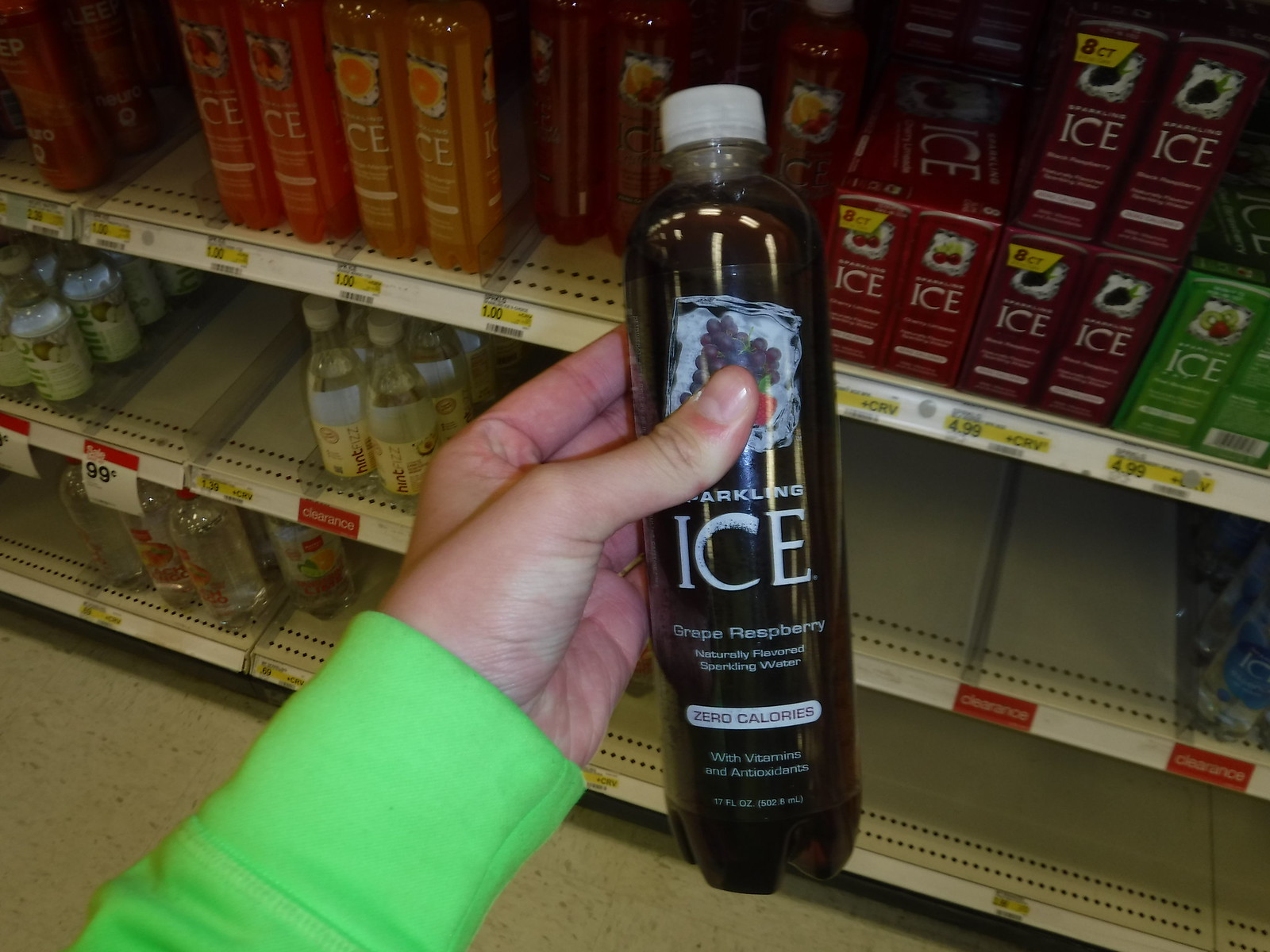The image depicts a woman holding a transparent bottle of Sparkling Ice grape raspberry flavored beverage in her left hand. The bottle, capped with a white top, contains a greenish-purple liquid and prominently features an image of ice, grapes, and watermelon on the label. Large white text spells out "Sparkling Ice" in the bottle's center, with detailed descriptions of the contents, including "grape raspberry naturally flavored sparkling water," "zero calories," and "with vitamins and antioxidants" below. Towards the bottom, the label notes the bottle size as 12 fluid ounces. The woman, wearing a green long-sleeved sweatshirt, has her thumb over the logo while her fingers wrap around the back. The background reveals department store shelving with cases and single bottles of Sparkling Ice beverages, along with visible price tags, signifying a grocery store setting.